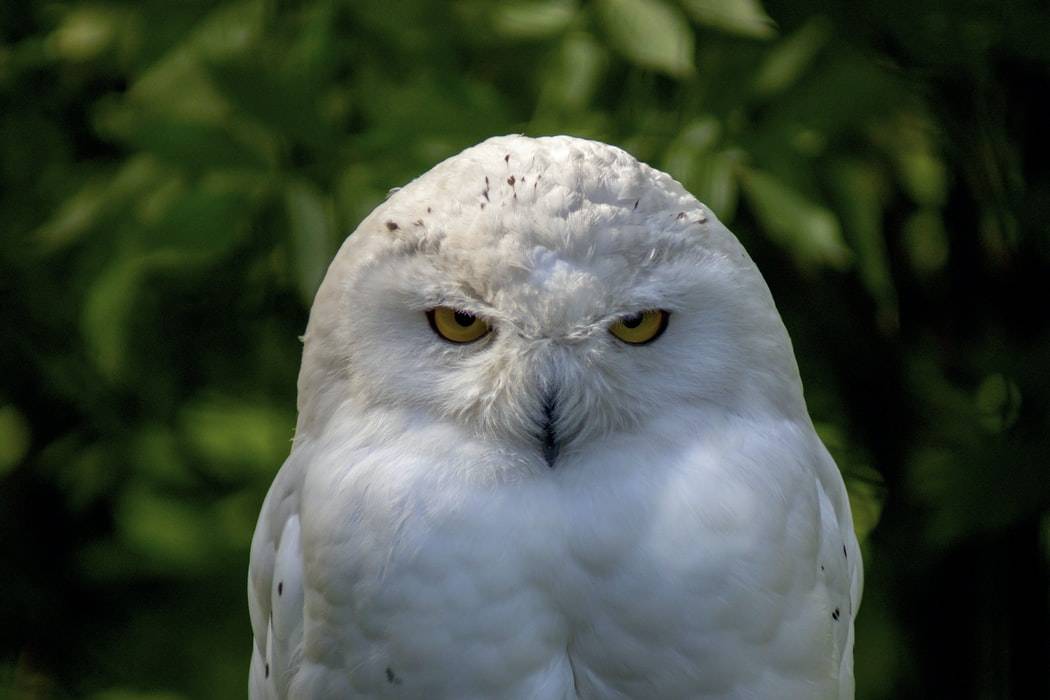This is an up-close, crisply detailed photograph of a snowy owl, which stands out in sharp relief against a blurred background of green vegetation. The snowy owl's bright white plumage is accented with a few black or brown flecks on its head and wings. Its eyes are a striking yellow, framed by bushy feather "eyebrows," and they stare directly ahead with a serious, almost angry expression. The owl's small black beak is partly obscured by feathers, and the individual feathers are so sharply captured that you can almost see each one. The center-focused owl's chest is puffy and white, adding to its full and fluffy appearance. The blurred background, with indistinct dark green leaves, emphasizes the clarity and detail of the owl at the forefront, making it the undeniable focal point of this well-composed photograph.